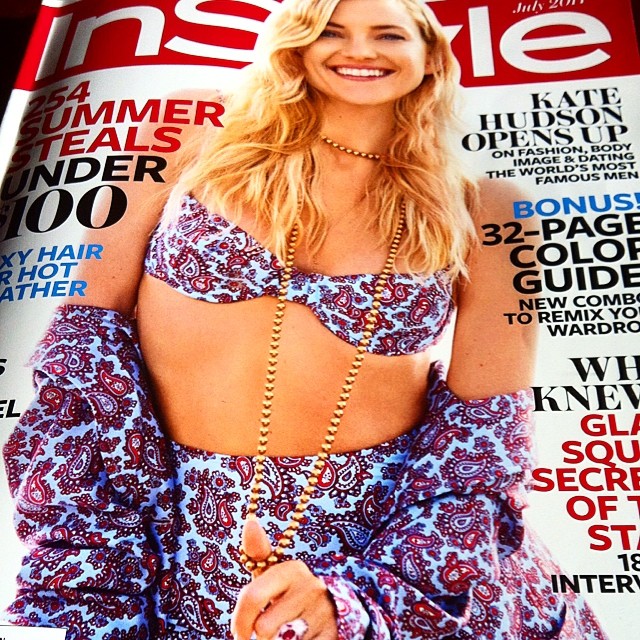The magazine cover features actress Kate Hudson with a radiant smile and long blonde hair. She is prominently displayed wearing a paisley-themed ensemble consisting of a long skirt, a matching bralette, and a light blue and red jacket, casually draped off her shoulders to reveal her bare shoulders. Around her neck, she wears a gold beaded necklace, which she holds with one hand, her thumb extended outward. The title "InStyle" is prominently written in white letters over a red banner at the top of the cover, partially obscured by her head. Above this, the date "July" followed by "2011" is visible. On the right side of the cover, text highlights include "Kate Hudson Opens Up on Fashion, Body, Image, and Dating the World’s Most Famous Men" and a bonus feature, "32-page Color Guide." Additional captions mention "240 Summer Steals Under 100," emphasizing the stylish and affordable theme of the magazine issue.